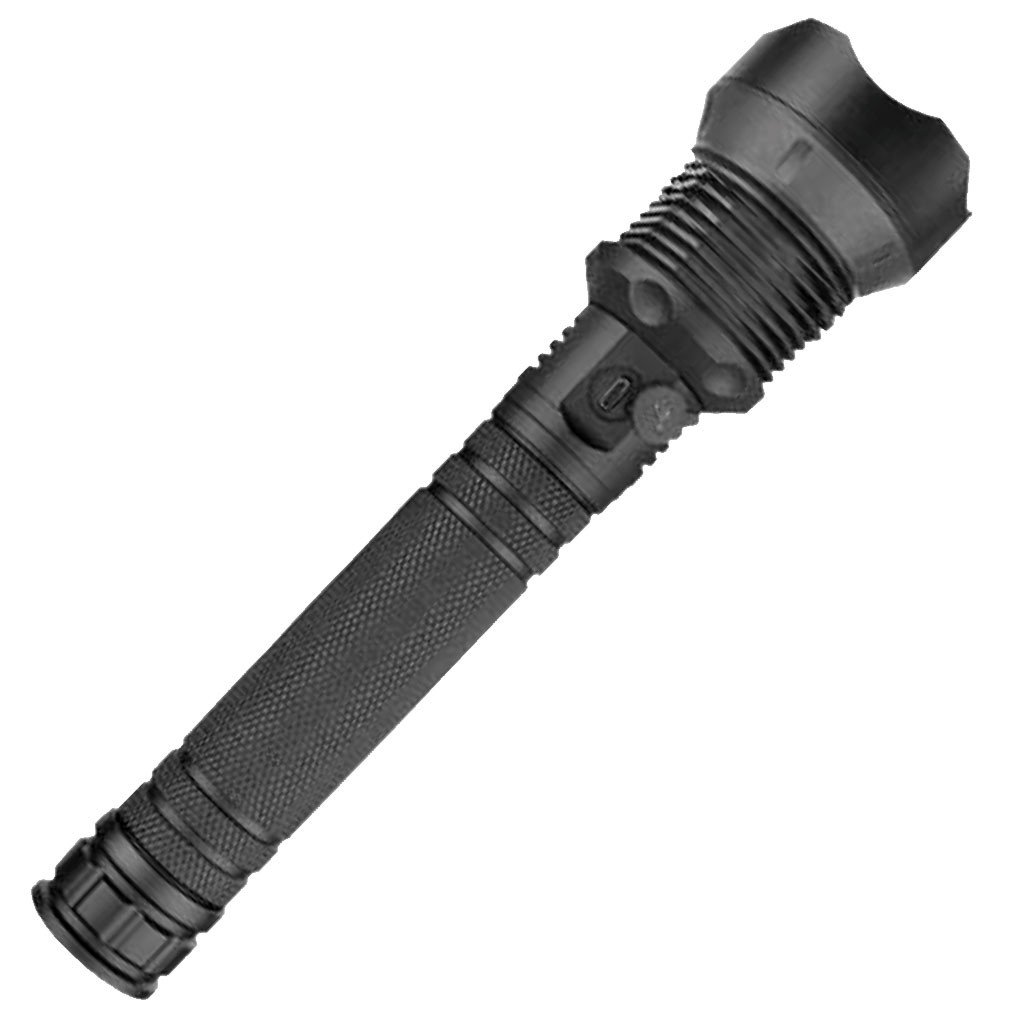The image depicts a heavy-duty, black tactical flashlight positioned diagonally on a plain white background. The flashlight extends from the upper right corner to the lower left corner of the image, with the top part larger and oval-shaped. Beneath the top, there are spiral details and textured indentations designed for a comfortable hand grip. The flashlight features a button and a USB port for recharging, indicating its rechargeable nature. There is also a bottom cap. The overall setup seems suited for a digital store display, emphasizing both the functionalities and the detailed design of the flashlight.